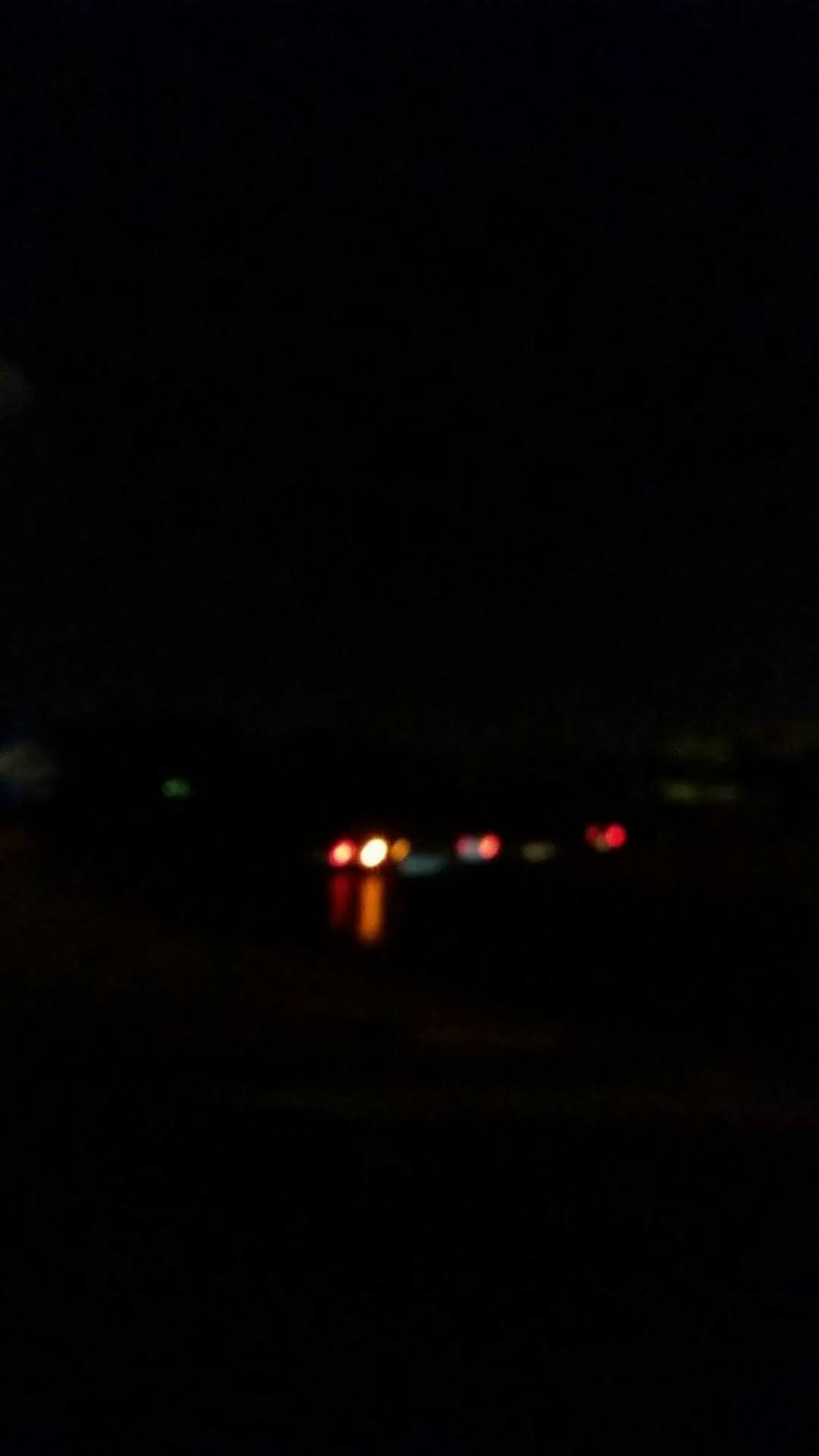In this very dark image, a structure that appears to be a bridge stretches horizontally across the middle of the frame, receding into the distance. The upper portion of the image is dominated by a nearly pitch-black sky, which enhances the nocturnal atmosphere. Despite the overall darkness, the bridge is discernible due to the vehicle lights that stand out, creating a glowing effect in the gloom. These lights, mostly red and white, dot the bridge and form a striking line that guides the eye across the frame. Most notably, two distinct reddish lights punctuate the left side of the bridge, adding a touch of color and depth to the otherwise shadowy scene.